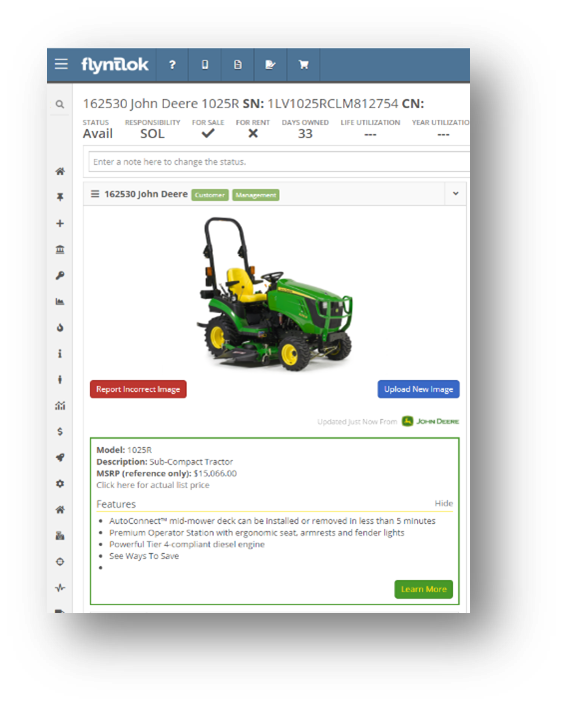The screenshot showcases the Flintlok website, spelled F-L-Y-N-T-L-O-K, dedicated to selling tractors and other farm equipment. At the top of the image, a blue horizontal bar spans the width of the screen, featuring the Flintlok logo with three lines on its left side. Centrally located within the bar are navigation icons, such as a question mark for help and a shopping cart icon.

Down the left side of the screen, there's a vertical gray navigation bar with black icons for various website sections, including a home icon for the main page, a bank-like icon presumably for financial services, several bar graph icons for statistical data, among other navigational sites.

Center screen, beneath the blue bar, black text details the item on sale: a John Deere tractor, model 1025R, with the product number 162530. Listed next to this is a serial number, indicating its unique identifier. The tractor is marked available with a checkmark next to "For Sale," and has been in ownership for 33 days.

Dominating the center is an image of the green and yellow John Deere tractor, a single-seater model. Below this image, a red box with white text says "Report Incorrect Image," while to the right, a blue box with white text reads "Upload New Image."

At the bottom of the page, a green-outlined box provides further details about the tractor, describing it as a subcompact model with an MSRP of $15,066. It boasts features such as Auto Connect and a powerful Tier 4 compliant diesel engine. Finally, at the very bottom right, a green box with yellow text invites users to "Learn More."